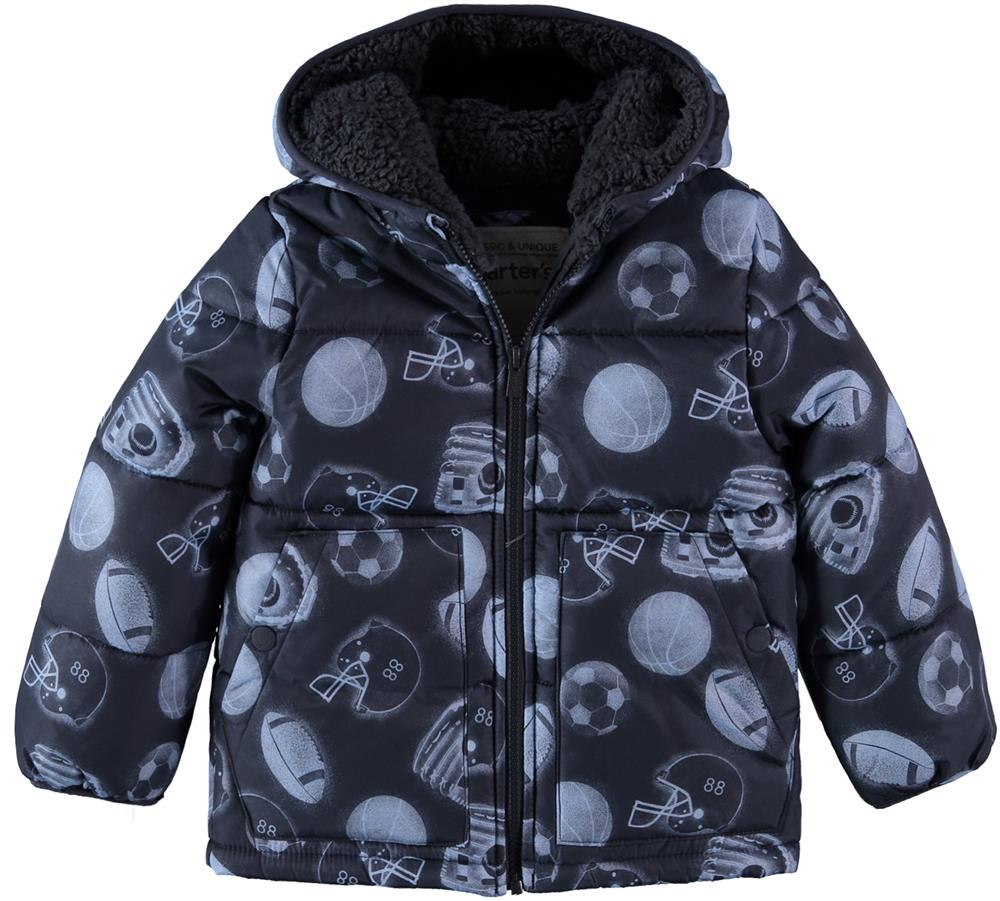This product photograph showcases a small child's puffy parka, designed with a black outer shell and black fleece lining inside the hood for extra warmth. The parka features a black zipper running down the middle, currently zipped up, and is adorned with a repeating pattern of semi-translucent white sports-related items. These items include baseball gloves with baseballs, basketballs, football helmets with white face masks and the number 88, black and white soccer balls, and white American footballs. The image, edited to have a flat white background, gives the parka a floating appearance, a common style for commercial photos typically found on online retail shops or in catalogs.